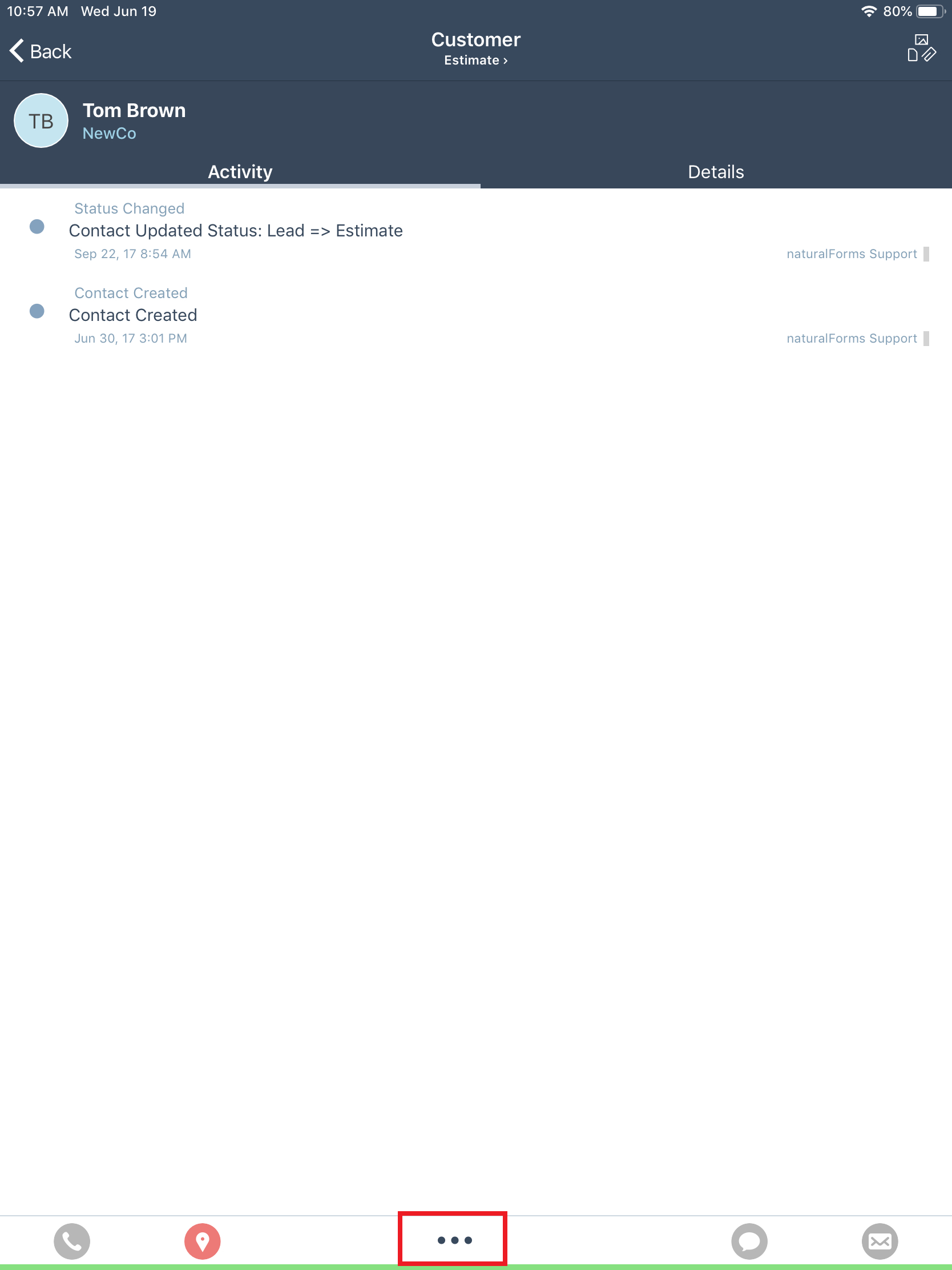In this image, set against a white background, we see a screenshot featuring a black header at the top. In the upper left corner of the header, white text displays the time "10:57 a.m." and "Wednesday, June 19th." On the upper right corner, a Wi-Fi icon and a battery icon showing 80% charge are visible. Below the time, an arrow pointing left is accompanied by the word "Back." Centered in the black header, white text reads "Customer Estimate."

Beneath the header, the name "Tom Brown" is displayed with a gray circle containing the initials "TB" to the left of the name. Below Tom's name, there are the words "New Company" followed by two tabs: "Activity" and "Details" with "Activity" being selected.

Against a white background and in gray text, further information is listed. The entry "Status changed, contact updated, status led = Lead = Estimate" is timestamped "September 22nd '17, 8:54 a.m." Below this, another entry states "Contact created" with the date "June 30th '17, 3:01 p.m."